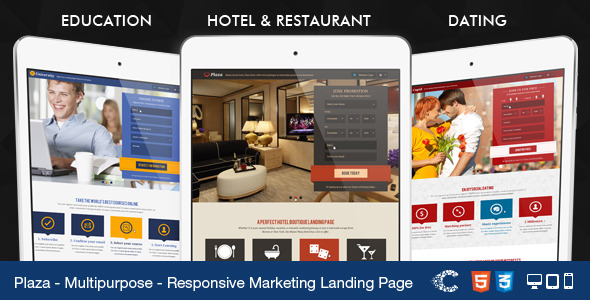In this visually captivating advertisement, three smartphones are prominently displayed, each showcasing a different scene to highlight diverse applications of a service. The first phone, labeled "Education," depicts a classroom environment where a young boy is seated at a table with a PC, although the image is somewhat blurry. The second phone, labeled "Hotel and Restaurant," reveals an elegant room furnished with a plush couch, a television, a stylish table, and sophisticated lamps, exuding comfort and luxury. The third phone, labeled "Dating," captures a romantic moment as a couple stands together; the woman is holding a bouquet of flowers, and the backdrop is adorned with a striking red and blue color scheme.

At the bottom of the advertisement, the text reads, "Plaza - Multi-purpose Responsive Marketing Landline," accompanied by a dissolving letter "C" resembling those effervescent pills that dissolve in water. Further down, the number "53" is displayed, along with icons representing a computer, tablet, and phone, denoting the cross-platform versatility of the service.